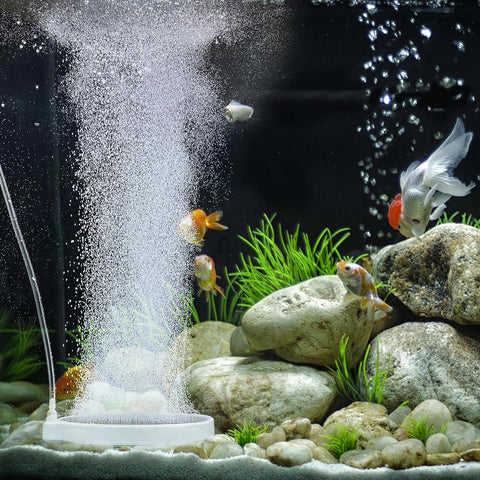The image depicts the interior of a square-shaped aquarium filled with colorful fish and a variety of underwater elements. The background is notably dark, highlighting a stream of fine bubbles rising from a white, circular aeration device located at the bottom left of the tank. This device is connected to a clear tube that extends upwards towards the upper right corner of the image. At the bottom, a layer of white sand slopes against the aquarium glass. To the right, a pile of rocks in pale and dark gray shades houses tufts of green plants poking through. Amidst the rocks and bubbling water, six fish of various shades of gold, white, orange, and yellow swim gracefully. Notable among these are a large goldfish, one with a prominent white tail, and a striking pure orange fish, all contributing to a vibrant and dynamic underwater scene.